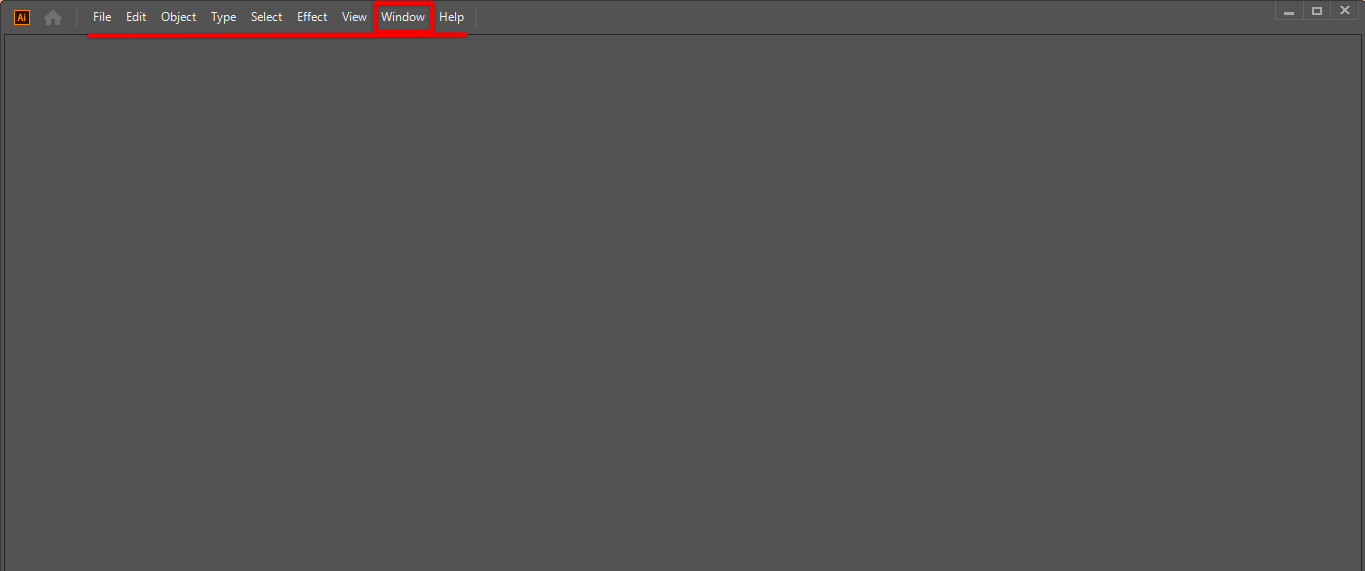The image features a stark, dark black background at the top. Prominently displayed at the center of this dark area is a red square with a black interior. Inside the square, the text "AI" appears in red, providing a striking contrast. Below this, there is a high-quality picture of a house, which draws the eye with its details.

Overlaid on the dark background are a series of white text options: "File," "Edit," "Object," "Type," "Select," "Effect," "View," "Window," and "Help." Each of these options is underlined with a thin red line, except for "Window," which is distinctively enclosed within a red rectangular box.

Positioned at the far right-hand side of the top section, there are three familiar buttons: a Minimize button, a square button that toggles full-screen mode, and an X button for closing the window.

Apart from these elements, the rest of the screen is completely empty, devoid of any additional content or interactive features.